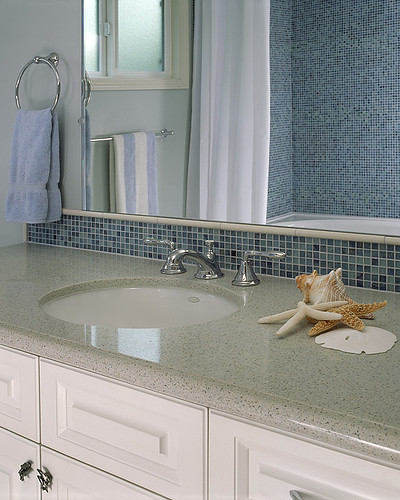In this detailed photograph of a bathroom, we see a pristine white vanity cabinet, adorned with a sophisticated, gray marble-look solid surface countertop speckled with black. The centerpiece of the countertop is a sleek, white round sink, paired with an elegant, large chrome faucet featuring widespread handles. Adding a touch of coastal charm to the scene are decorative items: an orange and white seashell and two starfish—one pale white and the other orange—gracing the countertop. The space is framed by a multicolored blue tile backsplash, creating a vibrant contrast against the white elements. 

Above the backsplash, a mirror hangs prominently, reflecting various details of the bathroom. A towel ring mounted next to the mirror holds a neatly hanging blue towel. In the mirror's reflection, a cohesive design theme is revealed with a towel bar supporting a blue and white striped towel, a closed window, and glimpses of the bathtub area. The bathtub features a white shower curtain and walls lined with matching blue tiles, subtly coordinating with the overall color scheme. The edge of the white tub can also be seen, contributing to the room's clean and inviting ambiance. The image is text-free, allowing the richness of the scene to speak for itself.